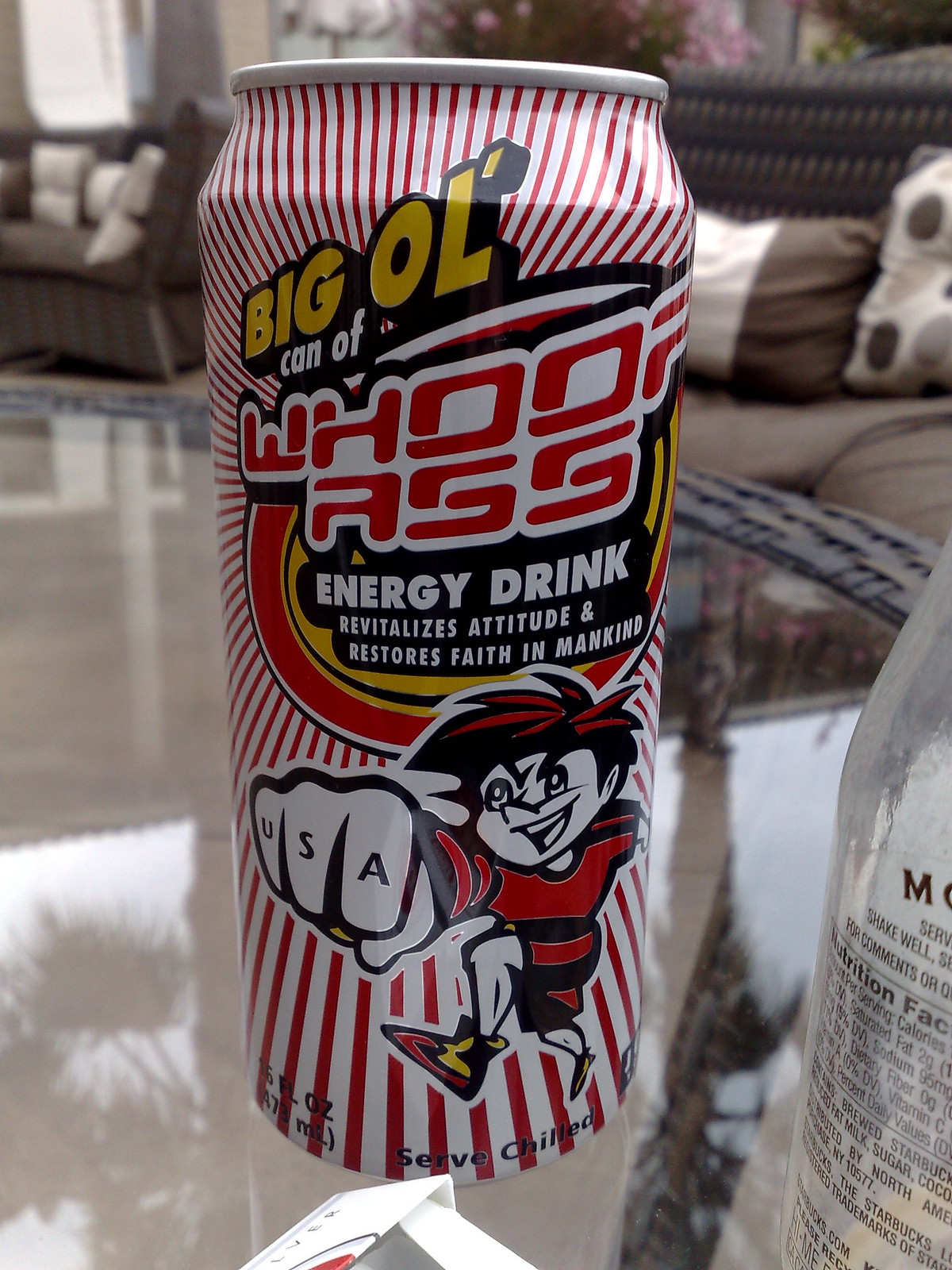The image features an aluminum can branded with the bold text "Whoop-Ass" across the front. The top of the can is adorned with dynamic red and white stripes that start from the top and bottom, converging into a prominent circular emblem. This emblem contains several words, reading "Big Old Can of." Beneath this emblem is an illustration of a boy with his fist extended, displaying "USA" written across his knuckles. The can rests on a round glass-topped wicker table. At the bottom of the image, there's a small box of cigarettes. To the right, an empty bottle is visible. The background showcases a wicker couch and another piece of wicker furniture, both featuring brown cushions.